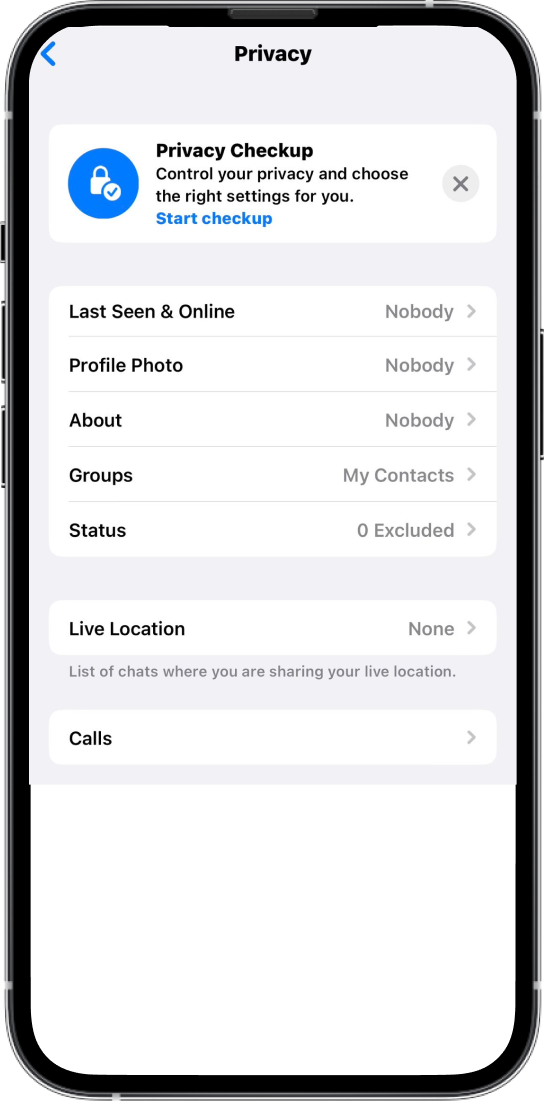The image displays the front screen of a smartphone, with a black border and curved edges around the glass. At the top, the word "Privacy" appears alongside a back button, allowing users to navigate to the previous screen. Below this, the heading "Privacy Checkup" is visible, followed by the text: "Control your privacy and choose the right settings for you," and a blue "Start Checkup" button. On the left side, there's a blue circle containing a check mark with a lock icon, indicating security features. To the right, an 'X' icon is available to close the message.

The screen is divided into sections against a gray background. The first section is a white box listing privacy settings:

- **Last Seen Online**: Nobody (with a right arrow for more information)
- **Profile Photo**: Nobody
- **About**: Nobody
- **Groups**: My Contacts (with a right arrow for more information)
- **Status**: Zero Excluded

A gray separator divides this from the next section, another white box, which includes:

- **Live Location**: None (followed by an explanatory text in gray: "List of chats where you are sharing your live location")
- **Call**: An option to click for more information

The overall interface is dedicated to managing privacy settings such as visibility of the last seen status, profile photo, and live location sharing.